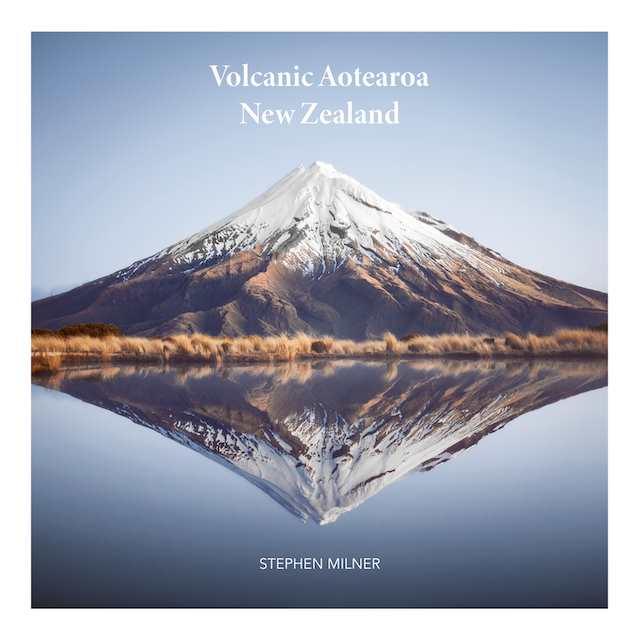The image is a striking photograph titled "Volcanic Aotearoa, New Zealand," prominently displayed in white font against a gradient blue sky. At the center, a small yet majestic volcano rises, its snow-capped peak standing in stark contrast to the rugged brown rock and grassland at its base. The surrounding landscape consists of tall, dry grass, suggesting a harsher, more arid environment. Below the volcano, a perfectly clear body of water mirrors the scene above, creating a flawless reflection that forms a diamond-like effect when paired with the mountain's peak. The artistically rendered photograph is credited to Stephen Milner, whose name is also in white at the bottom of the image.